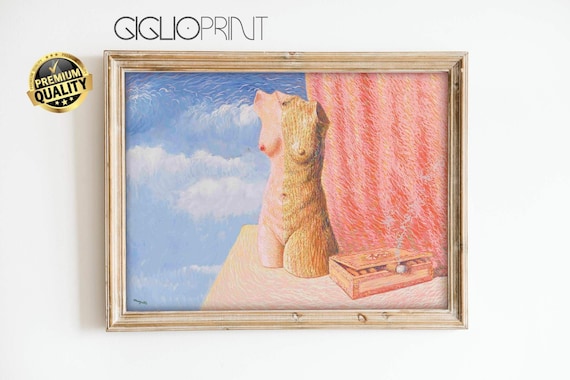The image presents a framed painting set against a gray background, labeled "Giglio Print" with a "Premium Quality" logo in a black circle with gold writing. The wooden frame encapsulates an intriguing and somewhat abstract depiction of a woman’s torso, displayed from the neck to the thighs, absent of head, arms, and legs. The left side of the nude torso features natural flesh tones, while the right side intriguingly adopts the texture and appearance of wood. Below the frame, a wooden box sits on a stand, with a single smoking cigar protruding from it, emitting a wisp of smoke. Adjacent to the torso, on the right, a red curtain adds a splash of color, contrasting with the sky and clouds visible on the left. The overall composition interplays elements of reality and abstraction, evoking curiosity and contemplation.